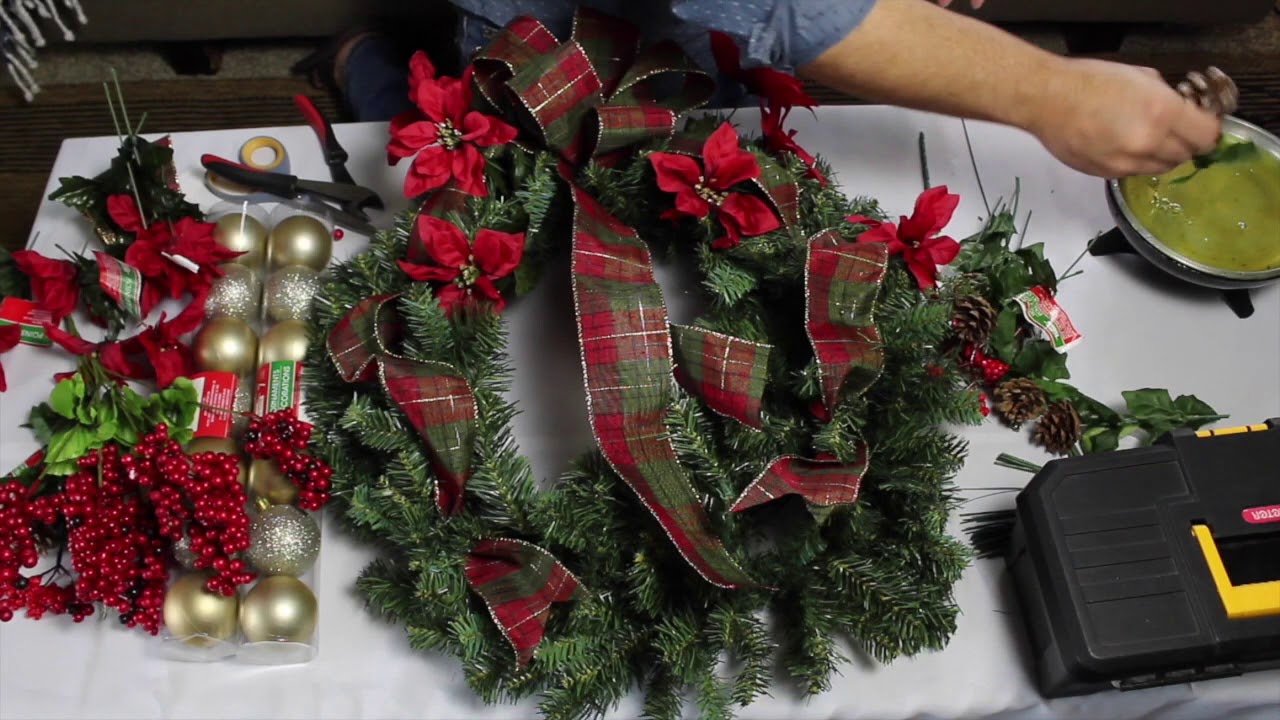The photo captures a detailed scene of someone engaged in creating a festive Christmas wreath on a white tablecloth-covered table. At the center of this horizontally oriented, rectangular image is a large, green wreath, approximately 18 inches in diameter, adorned partially with plaid red, green, and silver ribbons, and silk poinsettia flowers. The arm, presumably of a man, extends from the upper portion of the image toward the right, reaching for what appears to be a pine cone. Additional items, such as gold and silver Christmas ornaments, red berries with green leaves, and more ribbons, are spread out on the left side, awaiting incorporation into the unfinished wreath. A black plastic toolbox with a yellow handle sits in the lower right corner, accompanied by pliers, suggesting a hands-on crafting process. The entire scene is set on a white tablecloth, indicating a workspace dedicated to this creative holiday project.